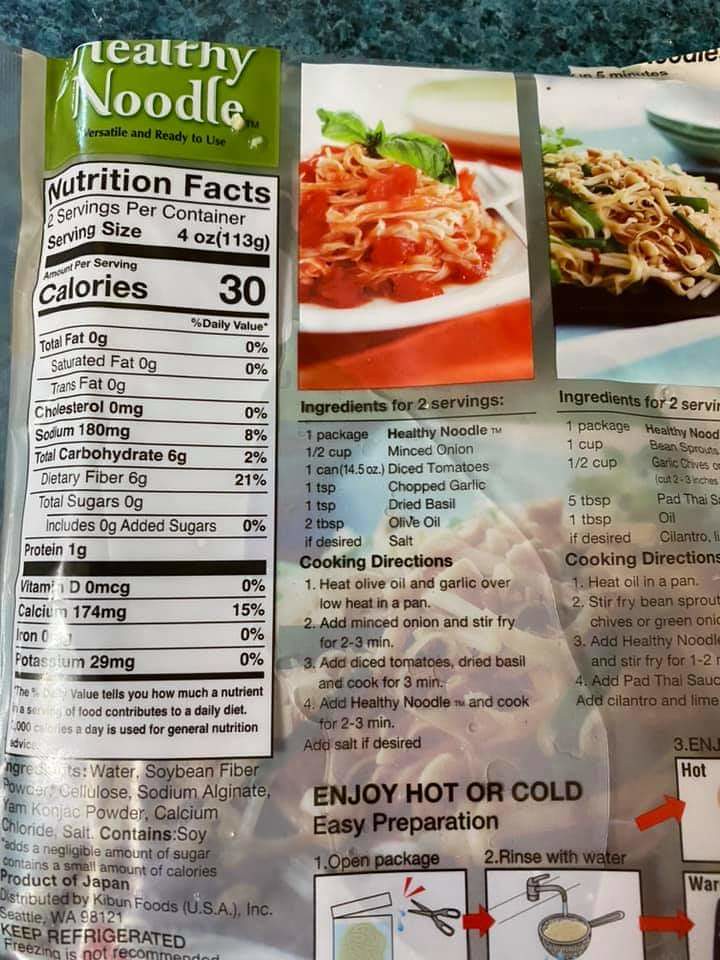This image shows the back of a packaged food product labeled "Healthy Noodle." The top section of the packaging features a green background with white text reading "Healthy Noodle" and just below it, in smaller black text, "versatile and ready to use." The top of the image also reveals part of a dark blue countertop, indicating the package has been opened.

Beneath the product name and description, the nutrition facts label provides detailed information about the food's nutritional content, including two servings per container, each serving being 4 ounces (113 grams), and a total of 30 calories per serving.

To the right of the nutrition label, there are two colored images depicting different noodle dishes. The left image shows a tomato-based pasta dish, while the right displays another noodle dish with a mixture of brown and white ingredients. Underneath each image are recipes or cooking instructions relevant to the dishes shown.

The lower section of the packaging contains the ingredients list against a gray background, followed by preparation instructions. The instructions emphasize that the noodles can be enjoyed hot or cold and outline a four-step process with white square icons and red arrows for clarity. The packaging indicates that the product should be refrigerated and mentions that it originates from Japan.